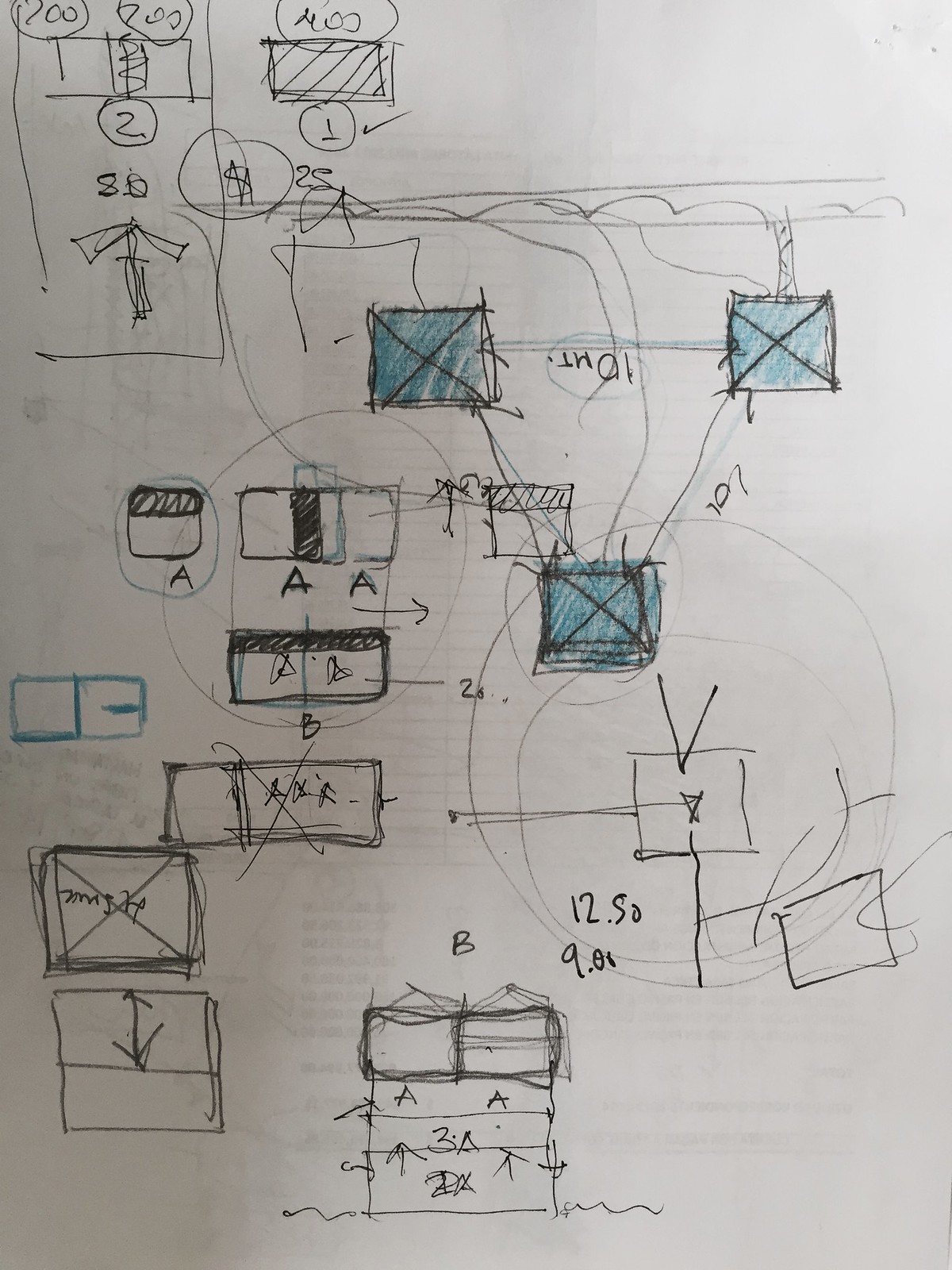This photograph captures a detailed drawing that resembles a schematic or a set of instructions. The illustration is rendered on white paper using either pencil or black pen for most of the content. Various alphanumeric characters and symbols populate the drawing, though they do not form coherent words.

Key annotations include:

- Items marked "A," "AXF," "3A," and "10MT."
- Blue or teal markings, characterized by squares with Xs through them.
  
At the top (presumably), a section includes:

- The number "400," both circled and accompanied by a rectangle underneath it, featuring a horizontal diagonal line. A circled "T" with a check mark sits beside it.
- Adjacent to this is another boxed entry, marked "200 200" with a circled "2" beneath it, but without a check mark.
- Additionally, a circled dollar sign is present on the page.

Overall, the drawing has a complex array of symbols and annotations, giving it the appearance of a technical, coded, or instructional document.